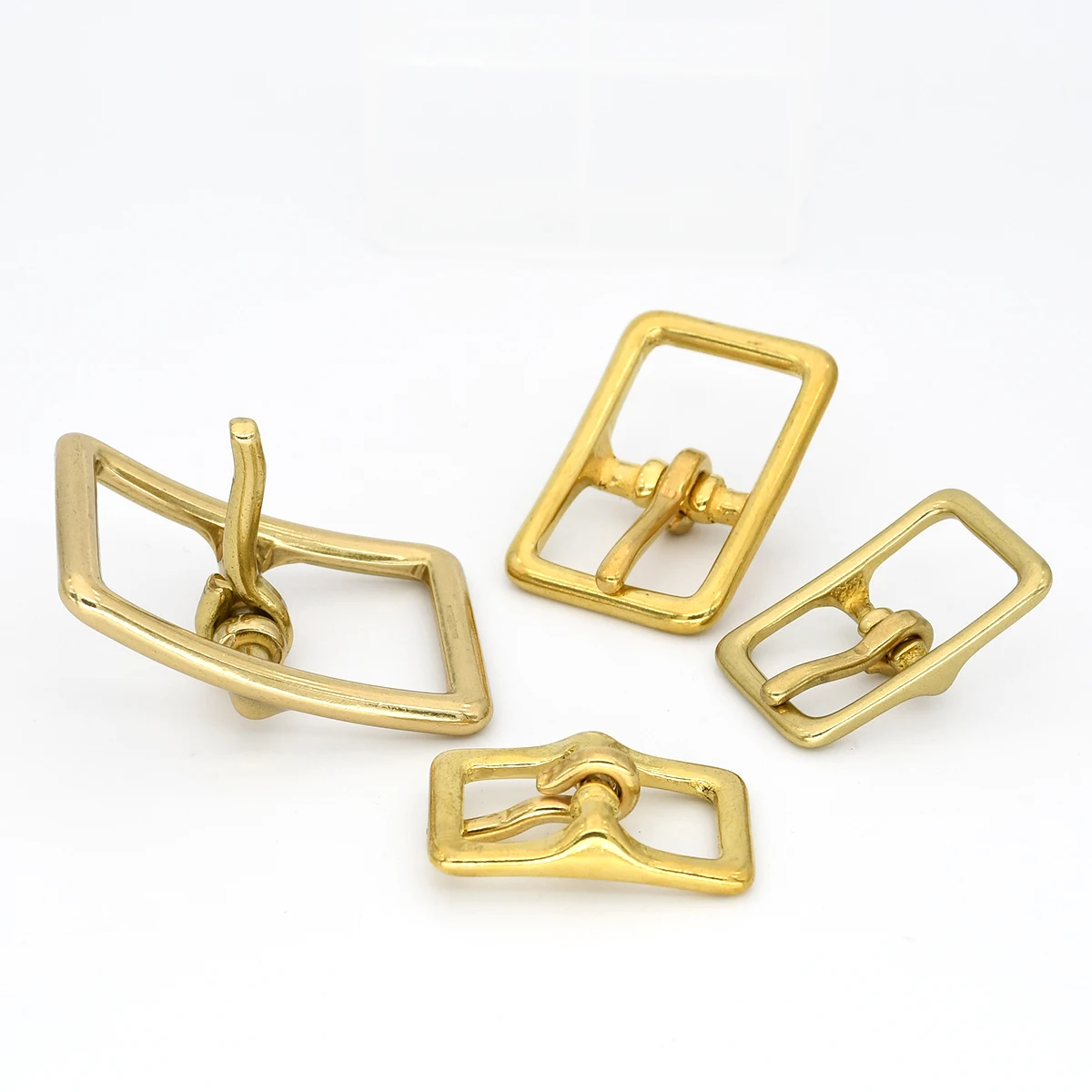This image features four shiny rectangular brass buckles of varying sizes, arranged on a seamless white background. Each buckle has a curved shape with rounded corners and includes a central metal prong for fastening. The buckles vary in brass tones, with two appearing warmer and two cooler. The largest buckle, positioned on the left, has its prong standing vertically, while the three smaller buckles have their prongs bent down flat. The smallest buckle is shown upside down, revealing the prong wrapped around the center bar. The scene appears professionally staged, reminiscent of a product photo for online sales, and the buckles include both bright and slightly worn finishes, highlighting their reflective surfaces.